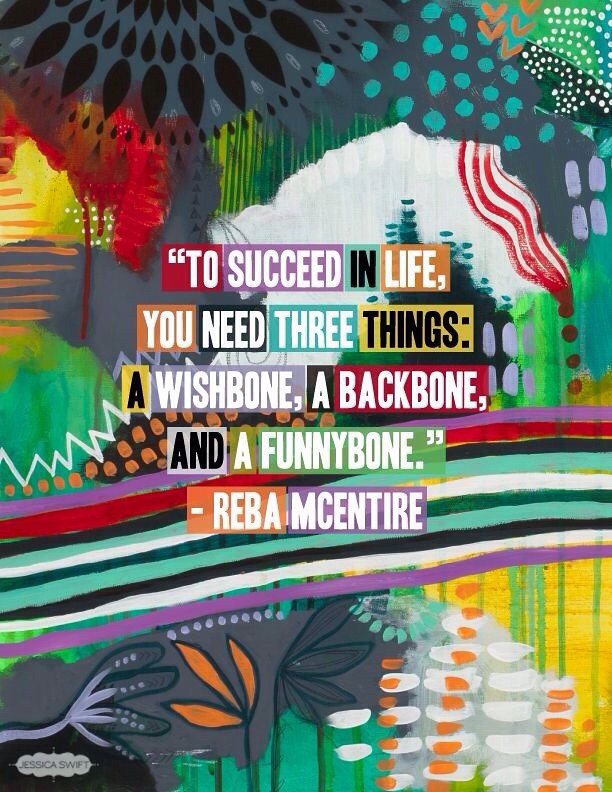The vibrant watercolor painting is a mesmerizing blend of colors and patterns. At the top, the right corner features green dot patterns while the left showcases leaf-shaped designs. Below these elements, various abstract shapes in orange, red, gray, green, and black occupy the middle of the image. Further down, a series of colorful lines stretch horizontally from left to right, transitioning through purple, red, black, green, white, dark green, light green, black, white, and purple. Flower patterns are scattered near the bottom of the painting, adding to its rich visual texture. Superimposed on this psychedelic backdrop, a quote stands out in predominantly white and black text: "To succeed in life, you need three things: a wishbone, a backbone, and a funny bone. - Rebec Massenter." The entire composition exudes a sense of vibrant, chaotic beauty, filled with organic forms and a vivid spectrum of colors.